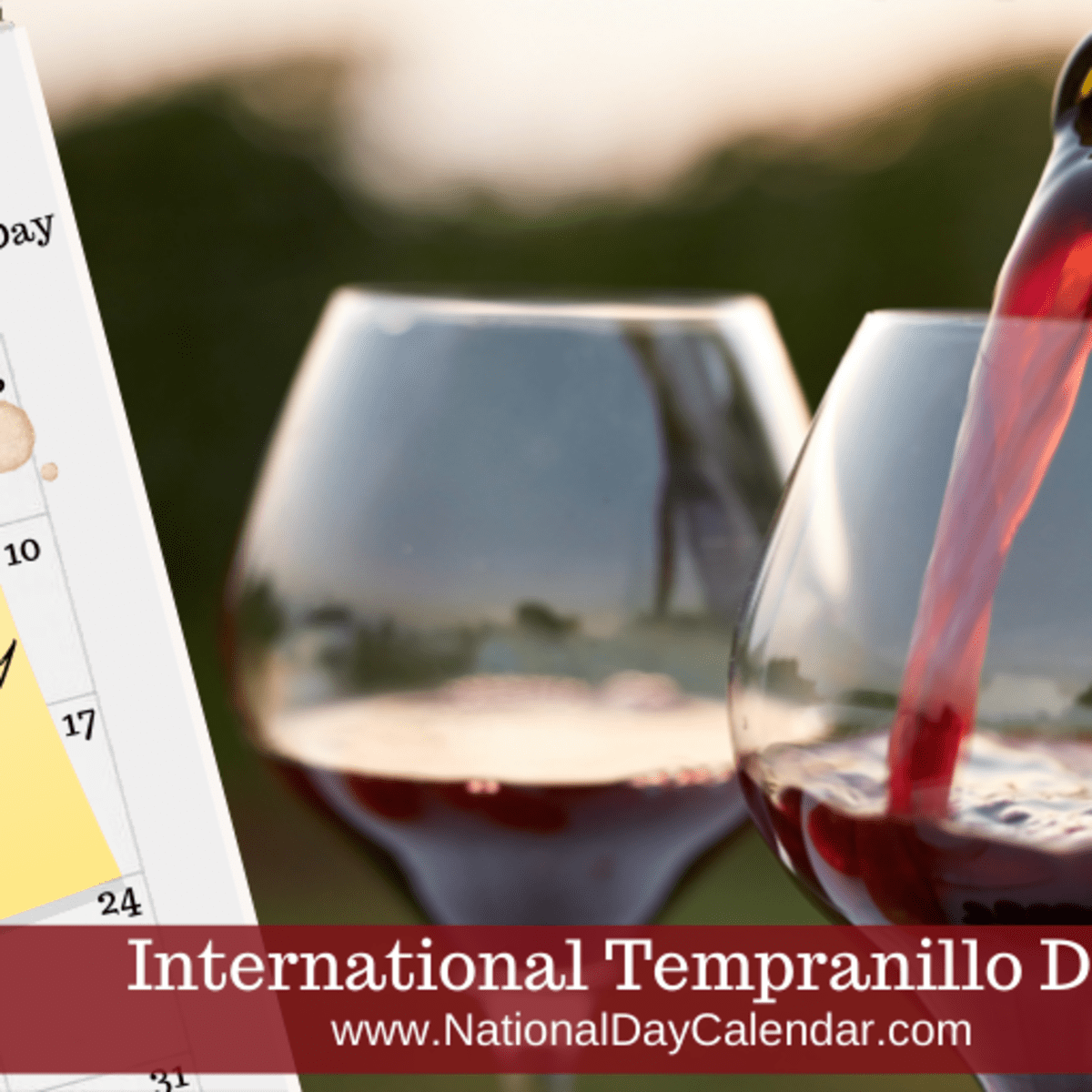The image is a close-up, color photograph in a square format featuring two large wine glasses side-by-side against a blurry background of green trees and a white sky, suggesting an outdoor setting. The wine glass on the left is about one-eighth full with red wine, while the glass on the right is being filled, with red wine pouring from a partially visible green wine bottle. In the foreground and overlapping the bottom of the image is a dark red banner with white text reading "International Tempranillo Day" and below that, the URL "www.nationaldaycalendar.com." On the left side of the image, partially out of frame, is a calendar showing the dates 10, 17, 24, and 31, with the word "day" visible at the top. The overall style merges photographic realism with graphic design elements.